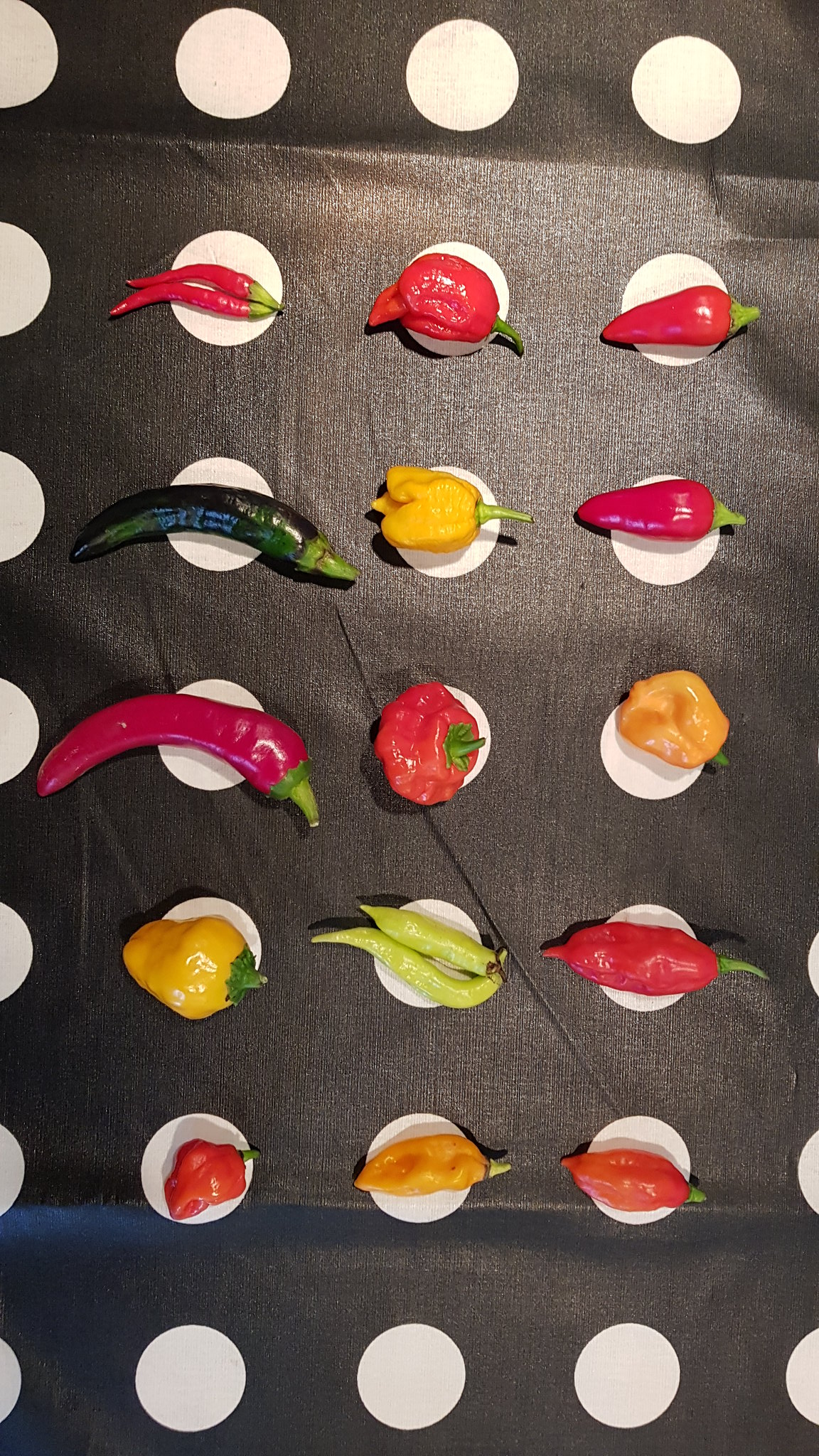In this color photograph, a variety of chili peppers are meticulously arranged on a black surface that resembles a tablecloth. The surface is adorned with a grid of 15 white, equally-spaced, flat paper circles. The peppers are positioned in three vertical columns and five horizontal rows, each pepper resting on one white circle. There are 15 peppers in total, showcasing an array of shapes and colors.

Starting from the top row, the leftmost pepper is a skinny, bright red one. The middle pepper in this row is plump, and the rightmost one is a traditional red chili shape. The second row from the top features a long, dark green, banana-shaped pepper on the left, a wrinkly, square-shaped yellow pepper in the center, and another traditional red chili pepper on the right.

In the third row, the leftmost pepper is a bright red, banana-shaped variety. The middle pepper is a very circular, wrinkly red one, while the rightmost is a small, yellow, wrinkly square-shaped pepper. The fourth row contains a yellow pepper that is fatter on top and thins out inwards on the left, a long, skinny, bright yellow-green pepper in the center, and an oval-shaped, wrinkly red pepper on the right.

The bottom row features a small, red-orange, wrinkly pepper on the left, a yellow-orange, slightly long pepper in the middle, and an oval-shaped, almost pink, red pepper with a little point on the end on the right. All the peppers retain their green stems, adding a cohesive detail to their varied forms and colors.